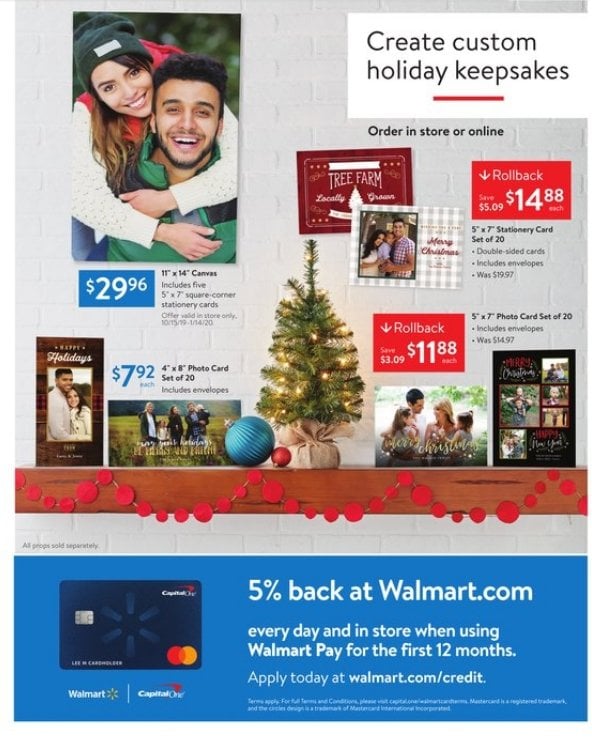The poster promotes the creation of custom holiday keepsakes, with a cheerful couple featured prominently on the left side. The woman is playfully riding on the back of the man, and both are laughing joyfully, capturing a moment of happiness. The background of the poster is a gradient of grey to white, giving it a clean and festive look. Accompanying the main text, which reads "Create Custom Holiday Keepsakes," is additional information stating "Order in Store or Online." The image is adorned with holiday elements, including a Christmas tree, enhancing the seasonal theme.